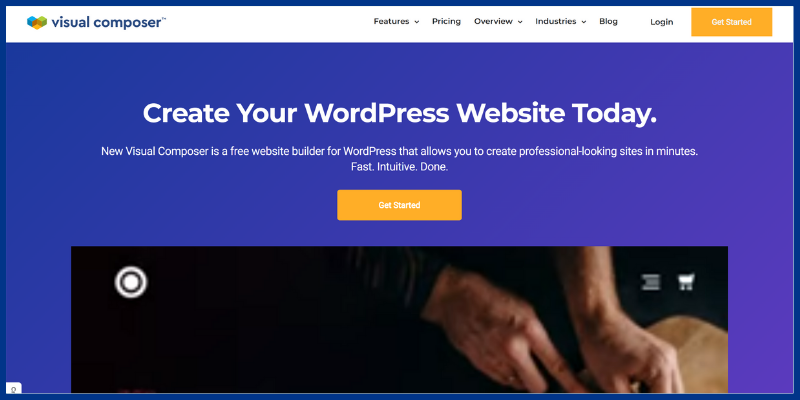The webpage features a vibrant gradient background starting with a medium blue at the top and transitioning to a purplish-blue towards the bottom right. At the top of the page, there is a white navigation bar with a distinctive logo featuring three cubes in blue, orange, and green on the left. The title "Visual Composer" is prominently displayed alongside a trademark symbol. On the right side of the navigation bar, there are several menu options, including "Features" (with a dropdown), "Pricing," "Overview" (with a dropdown), "Industries" (with a dropdown), "Blog," and "Login." An eye-catching orange rectangular button labeled "Get Started" is also present.

Beneath the navigation bar, the main heading in the gradient area reads, "Create your WordPress website today," with "WordPress" stylized as one word. Directly below, an introductory message highlights, "New Visual Composer is a free website builder for WordPress that allows you to create professional looking sites in minutes. Fast, intuitive, done." A prominent orange button beneath this text also displaying "Get Started" invites users to begin creating their site.

Additionally, about half of an image is visible below the text, featuring a close-up of a man's hands positioned over a cutting board. The specifics of the scene are obscured, with only the man's hands and the cutting board clearly depicted, leaving the impression that he is preparing food.